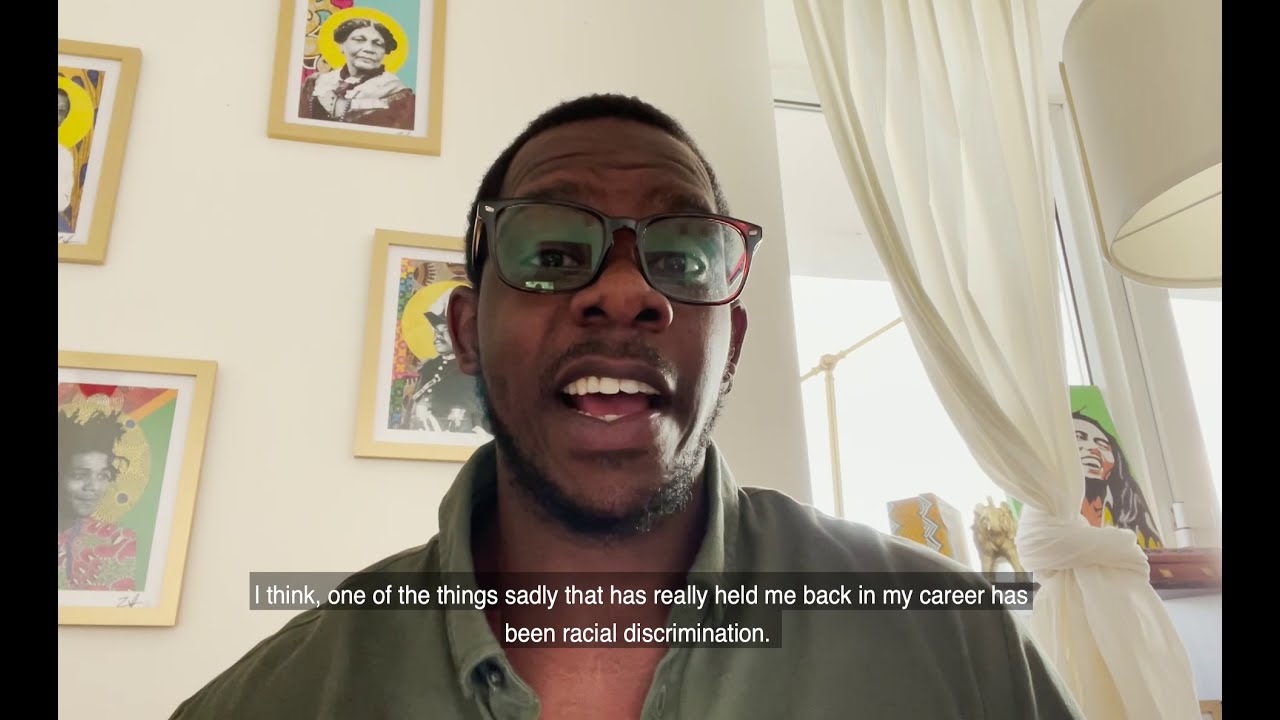The image features a black man seated centrally, speaking directly to the camera with his mouth open, revealing part of his tongue and teeth. He wears dark-framed, clear-lensed glasses, and has short black curly hair alongside a thin, neatly trimmed black beard following his jawline. He is dressed in a collared, button-up dark green shirt. Overlaying the image near his neck is white text that reads, "I think one of the things, sadly, that has really held me back in my career has been racial discrimination," indicating he is addressing issues of racism, likely in a video format.

The background is a white wall adorned with four picture frames, which seem to depict notable figures from black culture. To the right of the man, a white curtain is tied in a knot at the bottom, showing pronounced wrinkles. Next to the curtain is a window with a cloudy sky visible through it. Below the window sits a picture of Bob Marley with a greenish backdrop. Additionally, in the upper right of the image, there is a white cylindrical lampshade. The overall setting provides a sense of a personal, reflective space where the man discusses significant issues affecting his life and career.